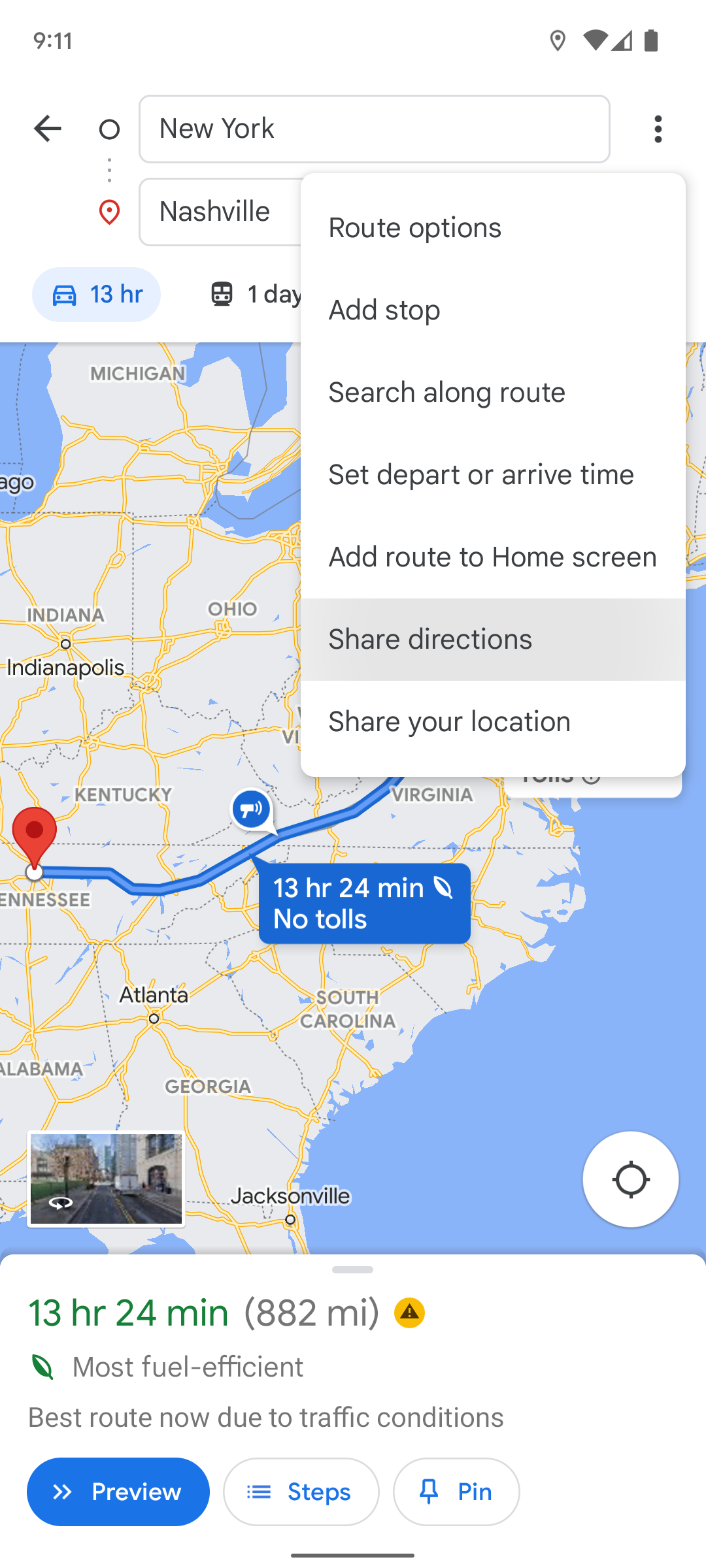A screenshot from a mobile device displaying a Google Maps navigation interface. The time in the top left corner reads 9:11. At the top of the screen, there are two boxes: one labeled "New York" and the other labeled "Nashville". A small car icon next to these boxes indicates a driving time of 13 hours. The main portion of the screenshot shows a map of the eastern United States, including a part of the Atlantic Ocean, with a blue route line stretching from New York to Nashville, Tennessee. The route is detailed with a note stating "13 hours 24 minutes, no tolls". Above the map, there's an option to "Share Directions". Below the map, highlighted in green text, the route details are repeated: "13 hours 24 minutes (882 miles)". Accompanying this are symbols including a circle with a black triangle and a leaf indicating "most fuel efficient". It then mentions "best route now due to traffic conditions". Further down, three oval buttons are visible: a blue one labeled "Preview", and two white ones labeled "Steps" and "Pin" respectively, the latter accompanied by a small push pin icon.